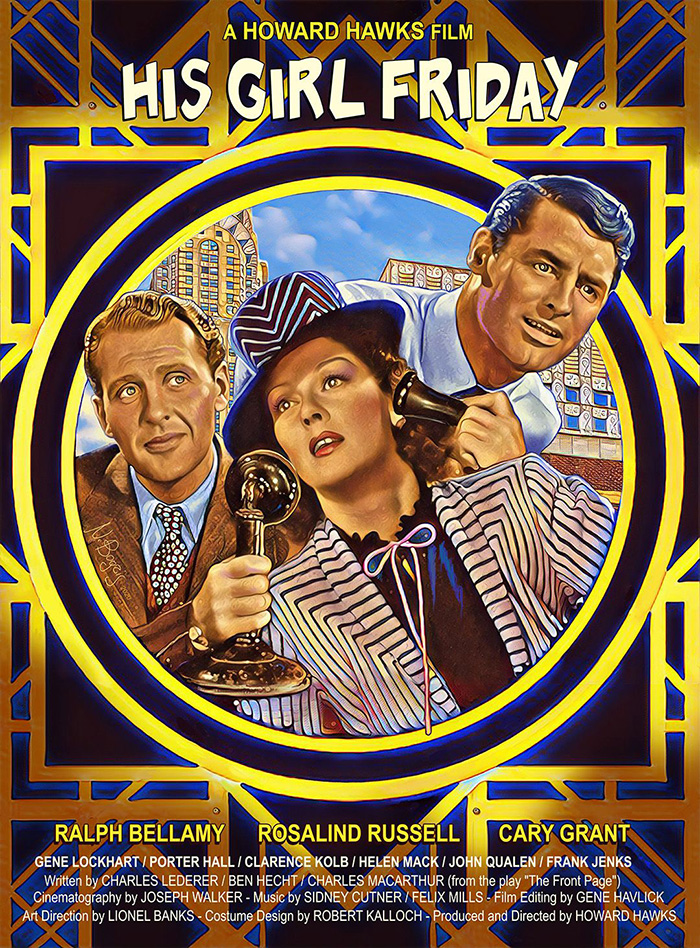This poster for the film "His Girl Friday," directed by Howard Hawks, features a central illustration of three characters, Ralph Bellamy, Rosalind Russell, and Cary Grant, dressed in 1950s or 60s attire, inside a circular cutout. The woman, presumably Rosalind Russell, stands in the center wearing a pinstriped suit jacket, a ribboned blouse, and a chevron hat, speaking into an old-fashioned rotary telephone. The men flank her: one in a three-piece suit looking in her direction, and another peeking from behind her. The poster's design includes a yellow circular frame adorned with various geometric shapes on a blue background detailed with yellow outlines. At the top, it prominently states "A Howard Hawks Film" in yellow, followed by "His Girl Friday" in an abstract, light yellow font. Below the illustration, the poster lists the actors' names and credits others involved in the film's production, such as writers and crew members responsible for cinematography, art direction, costume design, and production.